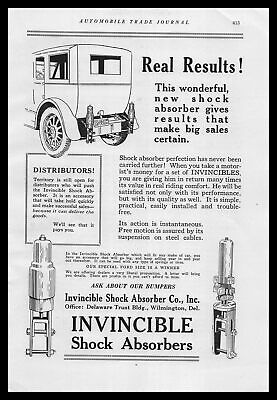This is a black-and-white advertisement clipped from an early 1900s trade journal, titled "Automobile Trade Journal," with a visible page number at the top and surrounded by a small black border. At the top, bolded text reads "Real Results," highlighting the benefits of a new shock absorber that promises substantial improvements in sales. The middle section features a very old-style automobile, reminiscent of a Model T, flanked by detailed descriptions of the shock absorber’s performance and distribution. Towards the bottom, the advertisement prominently displays images of the shock absorbers, described as "very tower-like looking," with a caption that reads "Invincible Shock Absorbers" and the company name "Invincible Shock Absorber Company Inc., Office Delaware Trust, Wilmington." All these elements are rendered in a distinctly black-and-white format, indicating the advertisement’s age and historical context.